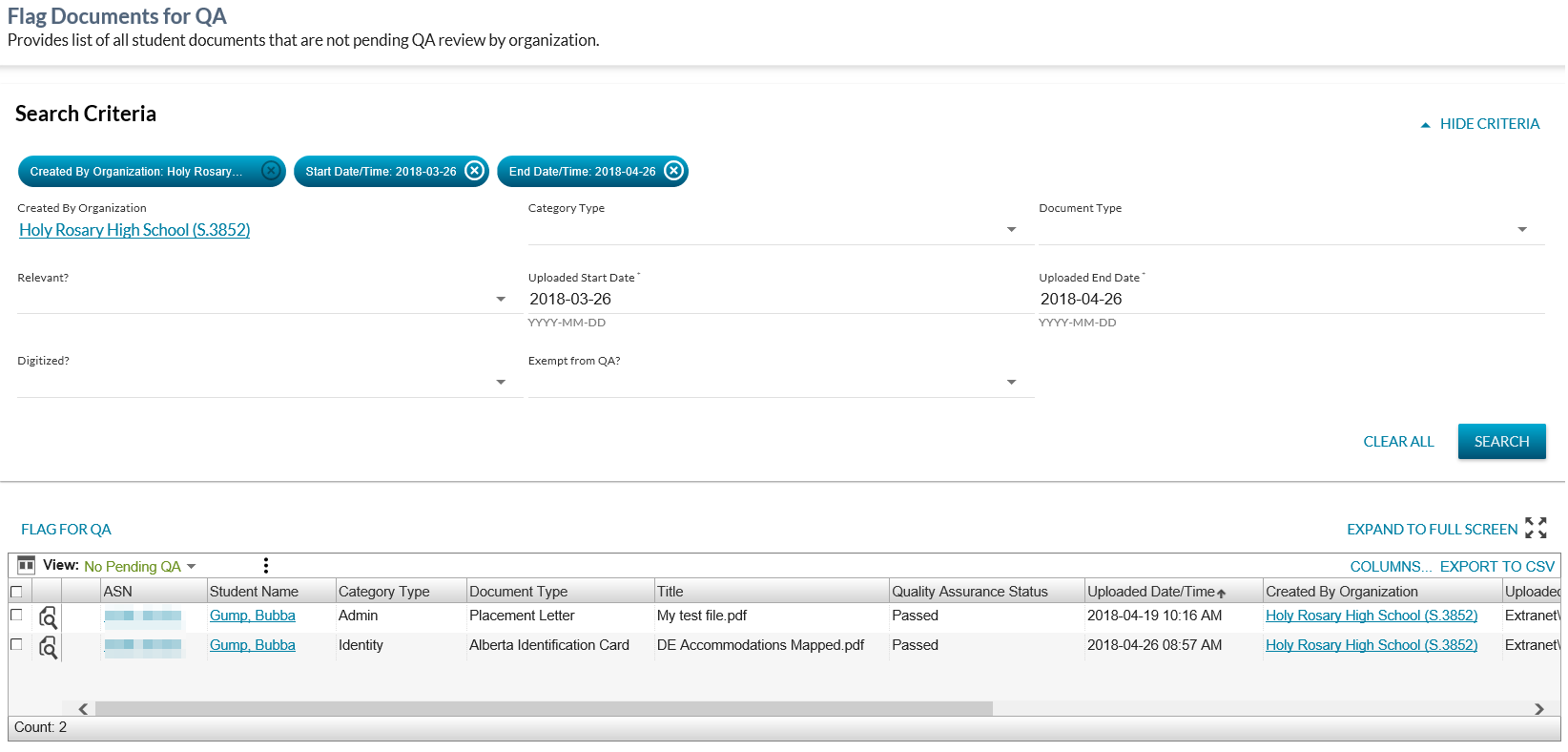Here is the cleaned and detailed caption:

"A cropped screenshot taken from a software application, possibly web-based or installed on a computer. The image highlights a specific section of the page dedicated to 'Flag Documents for QA.' The heading is followed by a subtext that reads, 'Provides lists of student documents that are not pending QA review by the organization.' The central portion of the image displays a search criteria area where a search has been conducted. Filter buttons at the top allow for refining or widening the search. The search parameters include a specific school, Holy Rosary High School, and set start and end times. The search results box shows two entries from the same student, indicating that there are no pending Quality Assurance reviews for these documents."